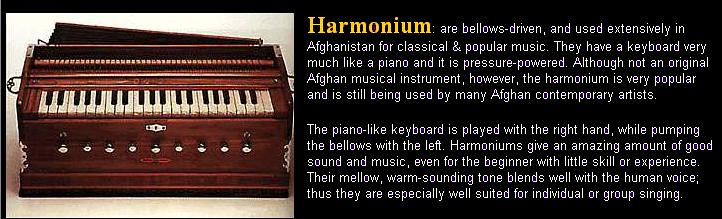This informational image features a detailed photograph of a harmonium—a bellows-driven, keyed musical instrument extensively used in Afghanistan for both classical and popular music. The instrument, appearing part organ and part accordion-like, is crafted predominantly from a rich brown wood, resembling mahogany. Its piano-like keyboard, comprising white ivory and black keys, is played with the right hand while the bellows, situated on the left, are pumped to generate sound. Several steel or silver pegs and multiple knobs adorn the wooden base of the harmonium. The instrument’s mellow, warm tones blend harmoniously with the human voice, making it particularly suited for singing, whether in solo or group settings.

The left half of the image displays the harmonium resting on an ivory or beige surface. The word "harmonium" is prominently highlighted in large yellow text at the top left, with the remaining description in white text on a black background filling the right side. The text explains that despite not being originally Afghan, the harmonium enjoys widespread popularity among contemporary Afghan artists. Its ease of use ensures that even beginners can produce good music, contributing to its enduring appeal in musical traditions.